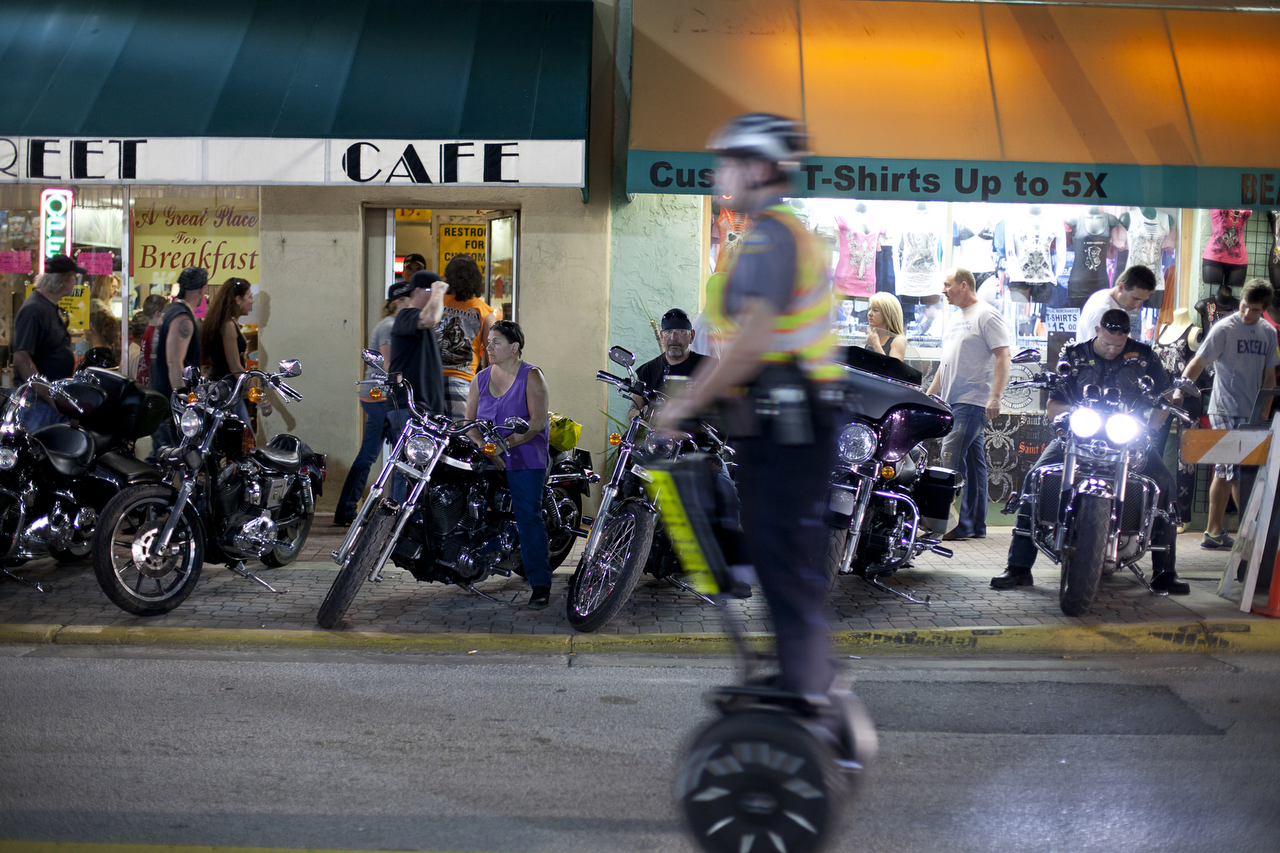The photograph captures a lively and somewhat amusing nighttime street scene. A police officer, dressed in a yellow jacket with reflective stripes, patrols on a two-wheeled scooter, reminiscent of a Segway, creating a humorous juxtaposition as he glides by a throng of rugged motorcyclists. These bikers, at least six in number, stand or sit on their motorcycles outside a street café and a custom t-shirt shop. The café, which advertises itself as "a great place to have breakfast," along with the t-shirt shop, casts warm lights onto the street, illuminating the gathering. The contrast between the officer on his modern, somewhat out-of-place scooter and the traditional, tough-looking bikers makes the scene both striking and amusing.